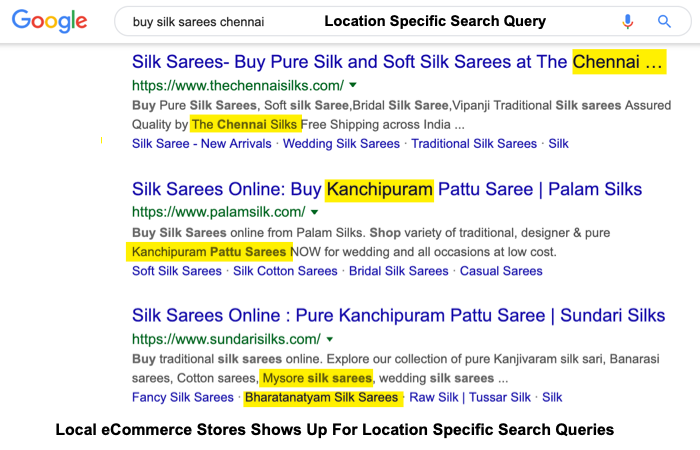This image highlights the results of a Google search for "Buy Silk Series Shaniai." The search results include three different links for purchasing high-quality silk sarees. The first link directs to ShaniaiSilk.com, offering a range of products including pure silk sarees, soft silk sarees, bridal silk sarees, Vipajan and Vipanji collections, and traditional silk sarees, all with assured quality and free shipping across India. The second result points to Palm Silks, where shoppers can buy a variety of traditional and designer silks, including pure Kanchipuram silk sarees, patu sarees, and options for weddings and all occasions, available at low cost. Additionally, they have selections of soft silk sarees, silk cotton sarees, bridal silk sarees, and casual sarees. The third link mentions Sundari Silks, another reputable place to purchase silk sarees.